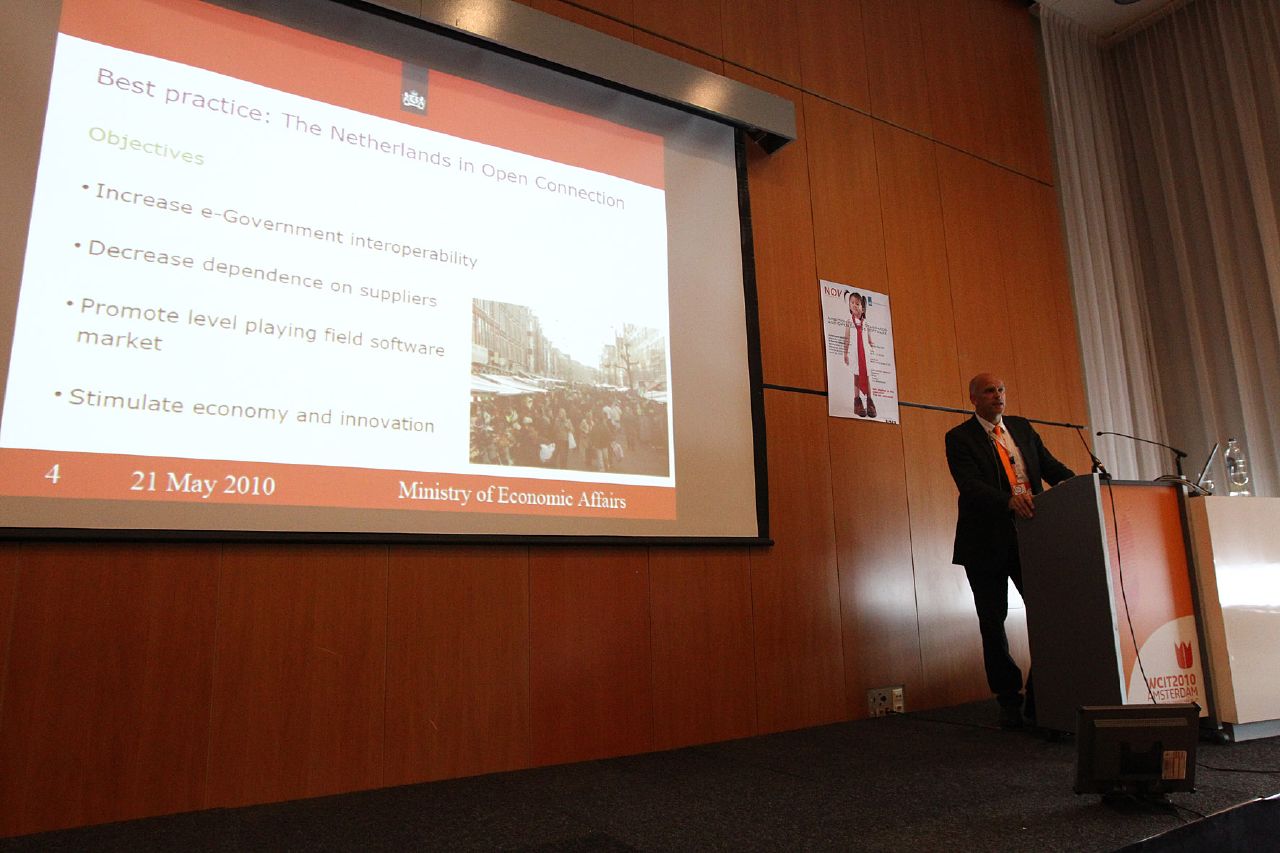This image captures a man, dressed in a black suit with a white shirt and an orange tie, standing on a dark gray stage behind a podium. The podium, positioned in the foreground on the right side of the image, features a gray side panel and an orange front panel adorned with a symbol at the bottom. Atop the podium rests a water bottle. The man is slightly turned to his right, addressing the audience through a microphone, indicating he is likely delivering a presentation or speech.

The backdrop includes a large screen displaying a presentation. Prominently, the slide reads "Best Practice," followed by "The Netherlands in Open Connection" and contains several objectives: "Increase e-government interoperability," "Decrease dependence on suppliers," "Promote a level playing field in the software market," and "Stimulate economy and innovation." At the bottom of the slide, it states, "21 May 2010, Ministry of Economic Affairs."

Behind the speaker is a brown wall with wooden panels and a white poster just above his head. To the right side of the background, there are tall, white, gauzy curtains covering what appears to be a floor-to-ceiling window. This detailed setup suggests a professional and formal conference setting, possibly WCIT 2010 in Amsterdam, based on the text inferred from the podium banner.